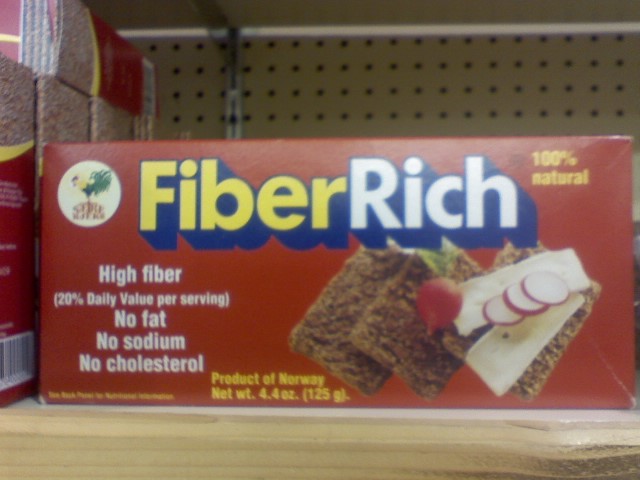This color photograph depicts a close-up of a box of Fiber Rich crackers positioned on a store shelf. The red, oblong packaging prominently features the words "Fiber Rich" with "Fiber" written in yellow and "Rich" in white against a large blue border. In the upper right corner, "100% natural" is written in yellow, and at the bottom, also in yellow, it states "Product of Norway, net weight 4.4 ounces (125 grams)". Below "Fiber" in the lower left corner, the text highlights "high fiber, 20% daily value per serving", as well as "no fat, no sodium, no cholesterol". The front of the box displays an appealing image of three crackers; one cracker is topped with two slices of cheese and three slices of radish, while a second cracker is decorated with a radish. Lastly, there is a small illustration of a rooster in the corner.